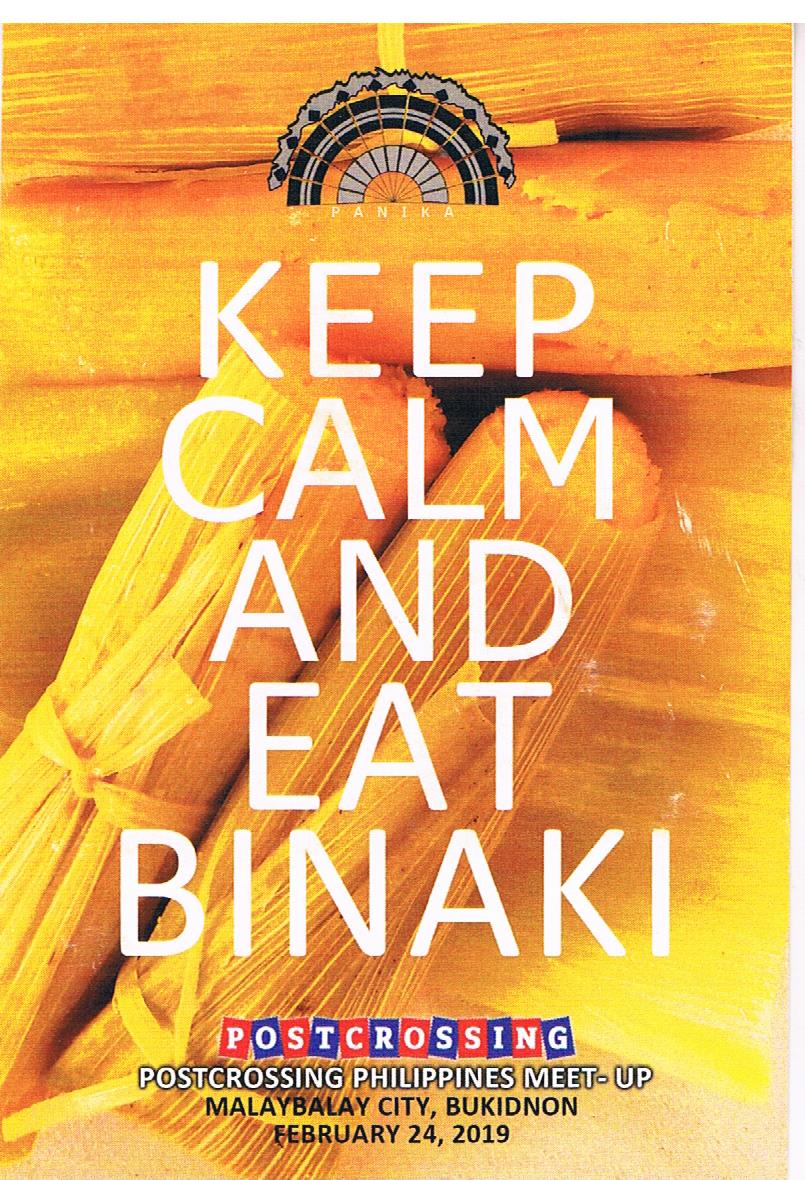The image showcases a promotional banner or poster predominantly featuring the phrase "Keep Calm and Eat Binaki" in large, bold white letters centered on a vivid, yellow-orange background. The backdrop is filled with images of tamale-like items wrapped in corn husks, presumably representing Binaki, a traditional Filipino snack. Also present is a symbol resembling a wheel, embedded within a section of gray and black hues above the main text. Beneath the central slogan, the poster details an event with the text: "Post-Crossing Philippines Meetup," further identifying the location and date as "Malabalay City, Bukidnon, February 24th, 2019." This combination of cultural imagery and event information clearly promotes a community gathering centered around the enjoyment of Binaki.